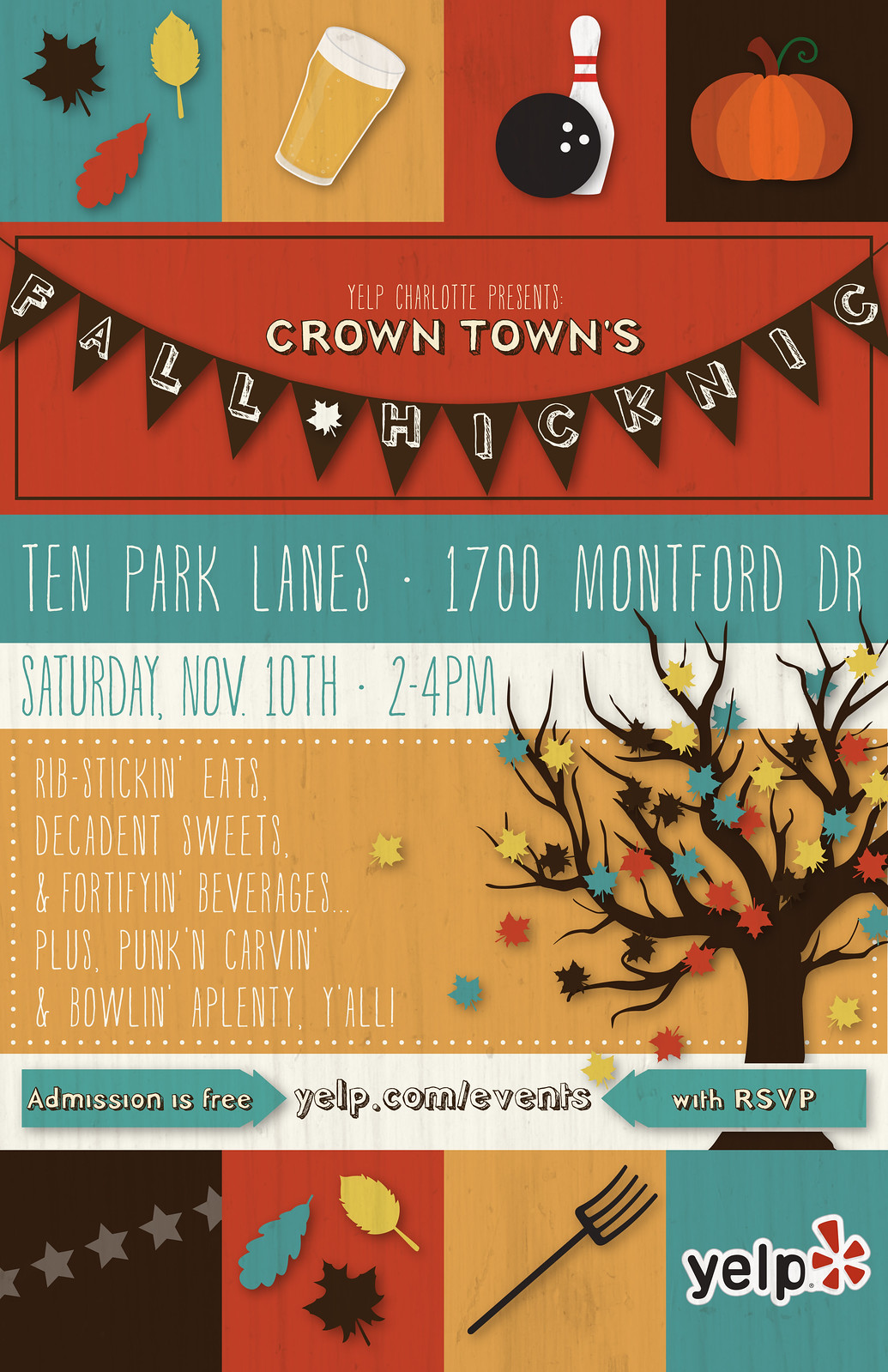This detailed poster, identified by its colorful and evocative layout, promotes Yelp Charlotte's "Crown Town's Fall Picnic." The top of the poster features a row of four vibrant squares: the first is turquoise with leaves, the second is beige with a glass of beer, the third is red with a bowling pin and ball, and the fourth is black with a pumpkin. Below these squares, a striking red rectangle displays the event's title, written on a banner: "Yelp Charlotte presents Crown Town's Fall Picnic." 

The event details continue in a blue rectangle that reads "10 Park Lanes, 1700 Montford Drive," followed by a white rectangle specifying, "Saturday, November 10th, 2 to 4 p.m." Further down, a yellow rectangle pictures a tree with colorful leaves and proclaims, "Ribs Stick'n Eats, Decadent Sweets, and Fortifying Beverages, plus Pumpkin Carving and Bowling Applenty, Y'all."

At the bottom of the poster, an invitation within a white banner states, "Admission is Free, Yelp.com Events, with RSVP." Finally, the bottom border mirrors the top with four equally sized squares: the first is black with stars, the second is red with colorful leaves, the third is brown with a pitchfork, and the fourth is turquoise featuring the Yelp emblem.